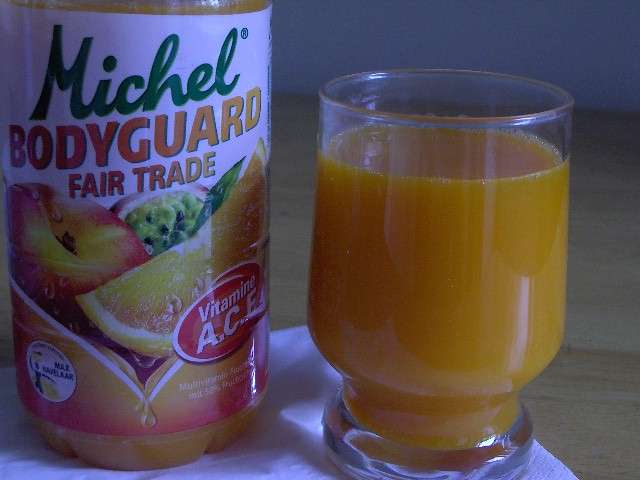The photograph captures a small, neatly arranged scene on a light brown Formica table, set against a plain white wall. At the center, a white napkin serves as a base for a deep orange juice-filled clear glass positioned to the right. To the left of the glass stands a bottle of juice. The bottle, containing an orange liquid, features a detailed white label. Prominent green letters spell out "MICHEL," and a yellow script declares "Bodyguard Fair Trade." The label also showcases images of an apple, an orange, and a piece of guava fruit, alongside an orange oval indicating the presence of vitamins A, C, and E. This nutrient-rich drink, appealingly presented, hints at a blend richer than simple orange juice.